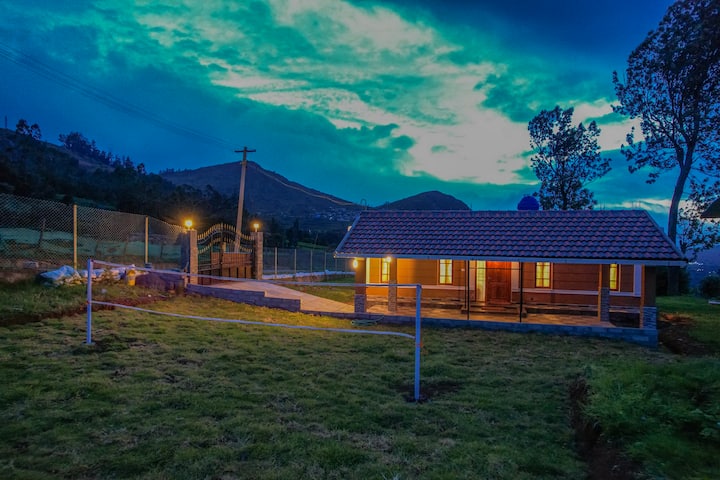In this uniquely colored photograph of a rural scene, a quaint, small house, radiating a warm glow, is featured at dusk. The house, with its brown wooden front, showcases a steep shingled roof that extends over a patio comprised of gray bricks, supported by wooden columns atop gray brick bases. To the left of the house, a sloped gray driveway leads to an arched metal gate flanked by gray brick columns, and a thin fence extends from the gate on either side. In the bottom third of the frame, a mown grass lawn dotted with brown patches appears, hosting a white badminton or tennis net near the bottom left.

The scene is set against a backdrop of rolling greenish-blue hills that gradually rise into towering greenish-blue mountains. Silhouetted power poles and power lines stretch from the upper left corner, leading towards the far center. The sky is an arresting mix of shades; while predominantly bright blue, it contains dark blue clouds in the top right and bottom left corners, with teal clouds gracing the center. Silhouetted tall trees populate the top right, adding to the serene atmosphere. Overall, the image harmonizes elements of rustic charm and natural beauty under a captivating evening sky.